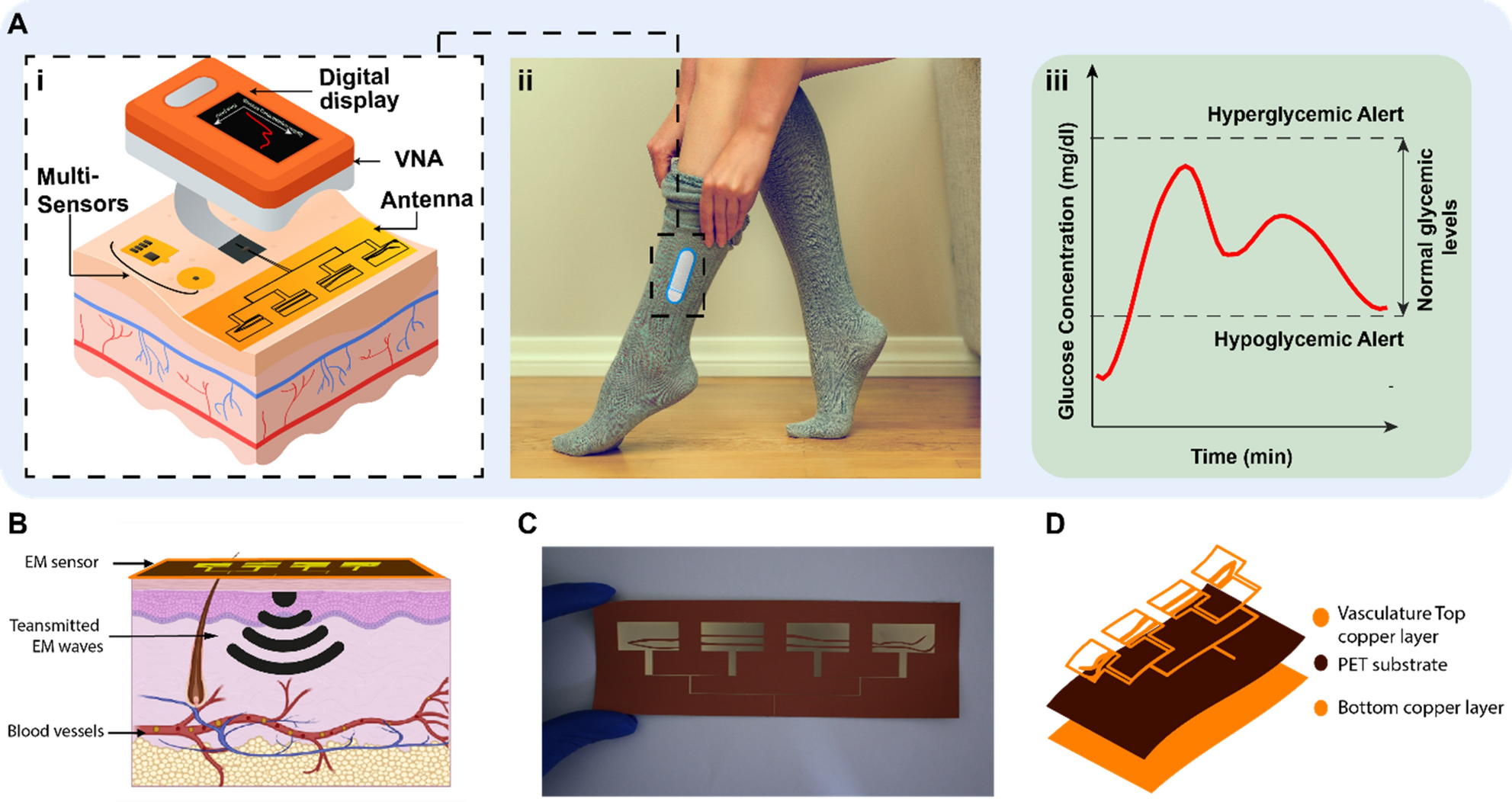The image is a detailed infographic divided into six labeled sections, organized in two rows. The top row, labeled as "A" with subsections I, II, and III, presents:
- **A1**: A tan cube device called a "digital display, VNA, and antenna" with multi-sensors and a yellow sticky note diagram. It's adorned with red and blue veins, highlighting its technological components.
- **A2**: A photograph of gray knee-high socks being worn by a person, showing a sensor embedded in the sock. The sensor is indicated by a white oval with a blue border, suggesting integration with the skin.
- **A3**: A graph depicting glucose concentration over time, marked with hyperglycemic and hypoglycemic alerts, and a red wavy line indicating varying glucose levels with normal glycemic levels annotated.

The bottom row, labeled "B," "C," and "D," provides further elaborate details:
- **B**: An illustration showing the epidermis with an EM sensor transmitting electromagnetic waves into the skin, reaching blood vessels.
- **C**: A close-up image of a person in blue gloves holding a brown rectangular sensor with four identical gold patterns.
- **D**: A cross-sectional diagram of the sensor device showing its internal layers – a vascular top copper layer, a PET substrate, and a bottom copper layer, each connected to the functions they perform in monitoring glucose levels.

Overall, the infographic showcases a comprehensive view of a glucose monitoring system designed to be worn within a sock, detailing its components, application, and the data it collects for monitoring blood sugar levels.